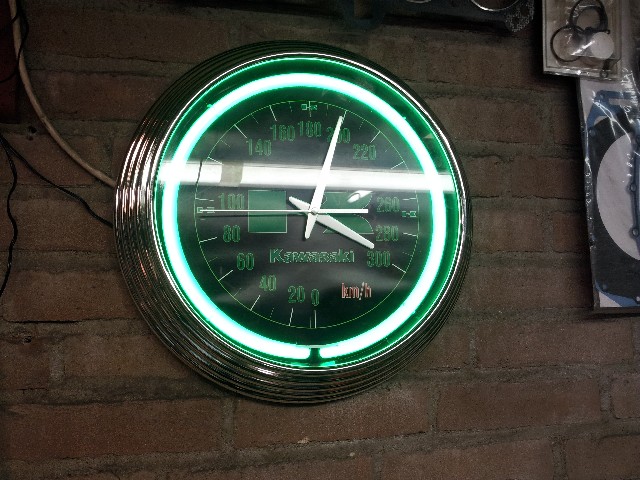In the image, a unique clock hangs on an aged brick wall. Designed to resemble a speedometer, the clock features a Kawasaki logo at its center and speed markings ranging from 0 to an unusual 300. The background of the clock face is illuminated with a vibrant green neon light, while a sleek chrome frame encases it. The clock's hands, including the hour, minute, and second hands, are all white, standing out distinctly against the green backdrop. Surrounding the clock, various elements are visible: cables, possibly providing power to the clock, extend towards the top left corner, and some items still wrapped in plastic occupy the top right corner. The brick wall itself is weathered, with mortar almost blending into the same color as the bricks, giving the setting a rustic and industrial appearance.